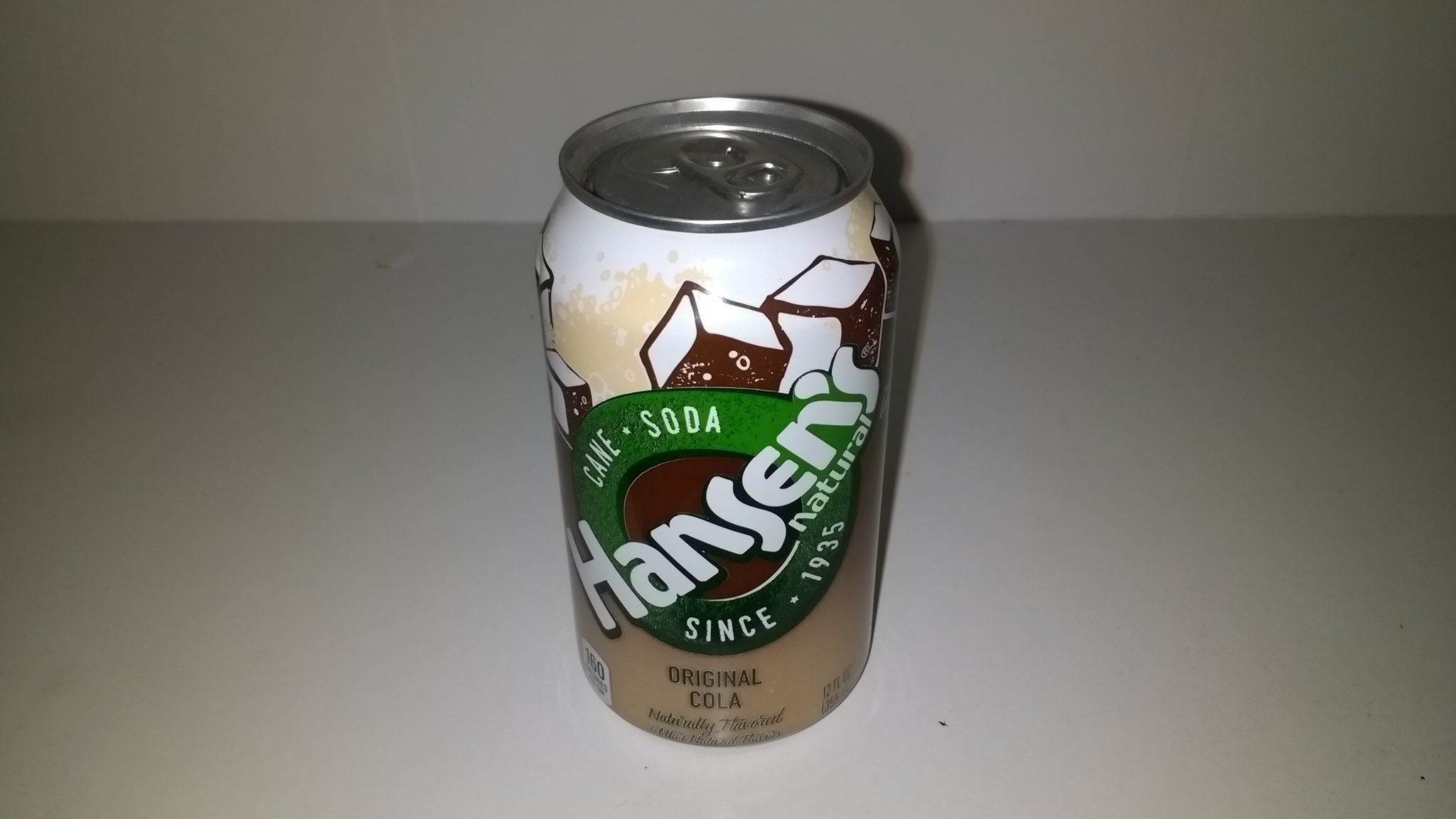The photograph is a horizontally oriented color snapshot, most likely taken with a flash, showcasing a 12-ounce aluminum can of Hansen's Natural Cane Soda, Original Cola flavor. The can is centrally positioned on a white surface against a white wall background. The design of the can features a gradient that fades from tan at the bottom to white at the top. Prominently displayed in the middle is a green circle with a brown center, which contains the white text "Hansen's" across the circle, and "cane soda" at the top, "since 1935" at the bottom. Below the circle, in black text, it states "Original Cola." Above the green circle, there's an illustration of brown and white speckled ice cubes on a beige and white background, emphasizing its naturally flavored cane soda. The can also has a metal top with a pull tab.